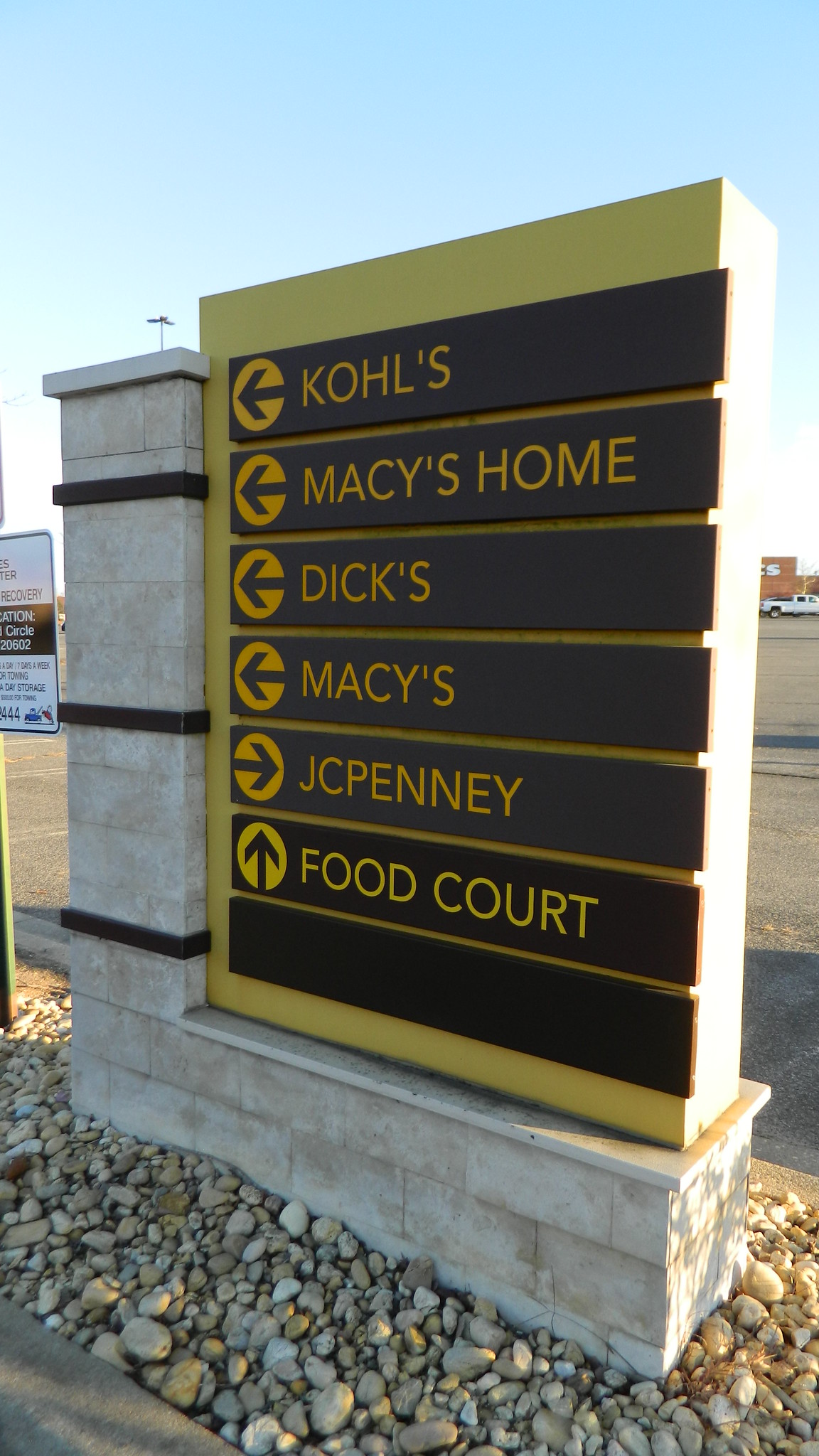This image captures the entrance of a shopping center, prominently featuring a distinctive sign. The sign is angled towards the lower left, supported by a unique L-shaped stone structure. The structure is predominantly white but features notable design elements: three brown circular patterns embedded in the stone. The sign itself is green and is complemented by several smaller signs attached to it. Each of these smaller signs lists the name of a store within the shopping center, along with arrows indicating the direction to each store. The base of the L-shaped stone structure also appears to have stone elements, providing a cohesive look to the overall design. The detailed craftsmanship of both the sign and its supporting structure emphasizes the aesthetic appeal often found in modern shopping centers.